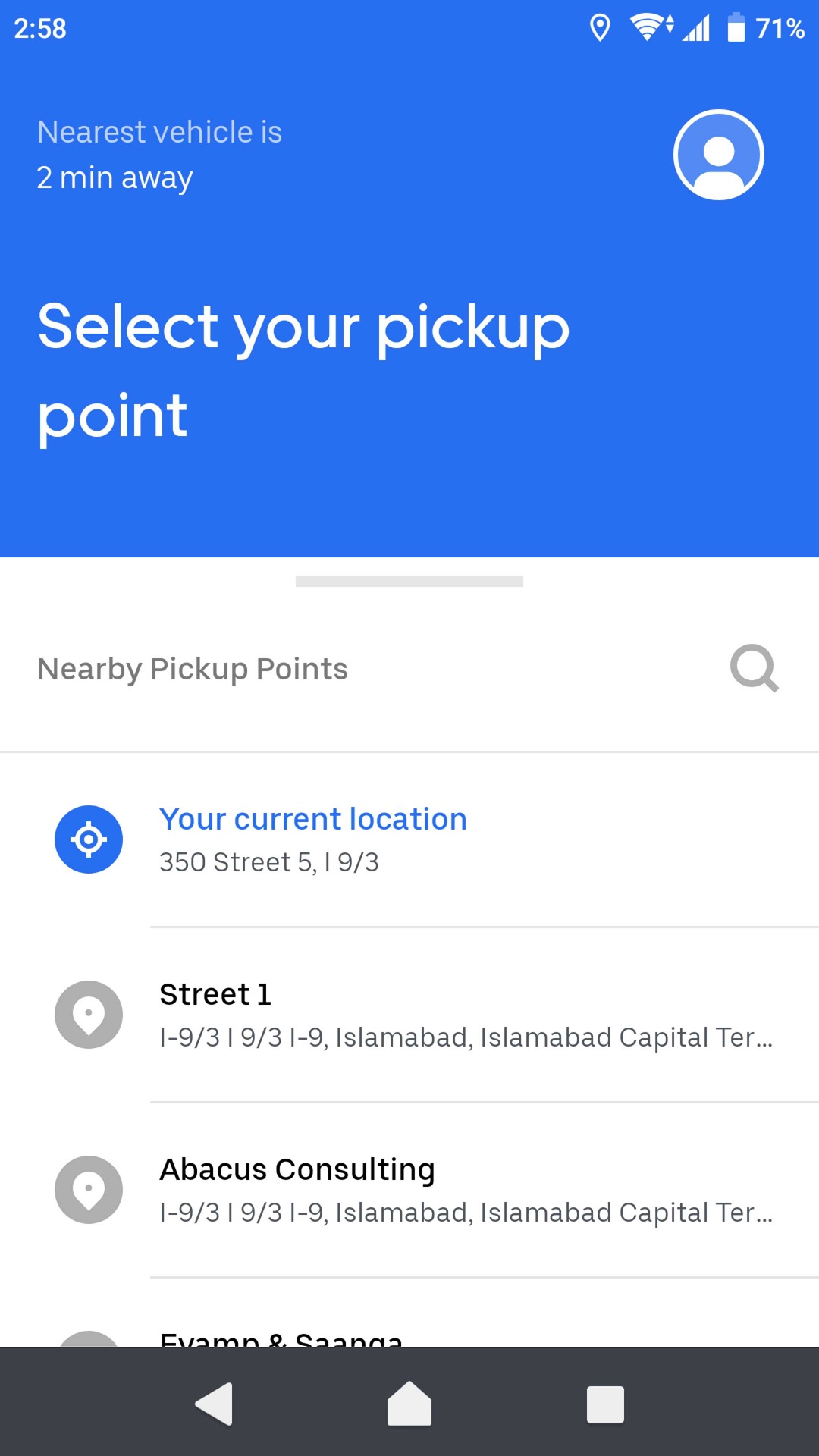This screenshot captures the interface of a ride-hailing app on a smartphone, displaying a 'Select Your Pickup Point' feature. The phone's status bar indicates the time is 2:58 PM, and the battery is 78% charged. The app is set to use the current location as the pickup point, specifically 350 Streets, a detail likely styled after Istanbul's geographical format. The visual theme and layout suggest the app is a Turkish version, akin to Uber, catering to users in Istanbul or a city with similar aesthetics.